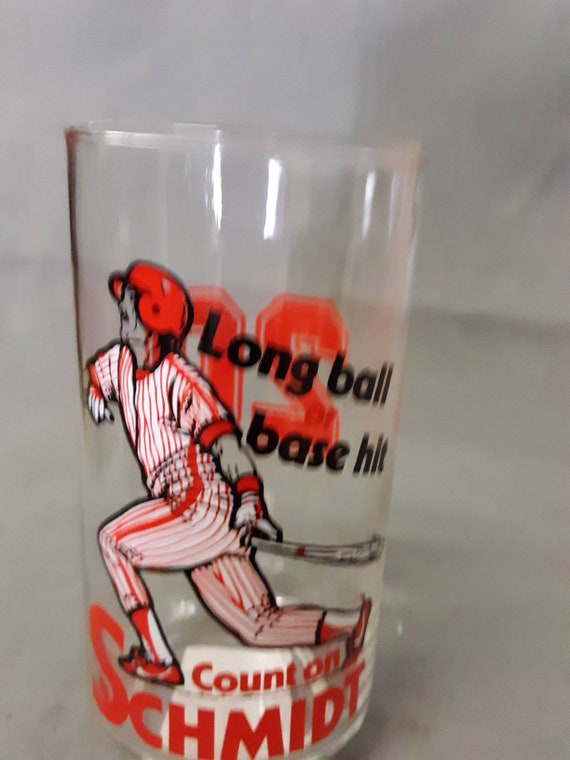This photograph features a clear glass, possibly plastic, showcasing a detailed illustration of a baseball player in motion. The player is wearing a red helmet and a red and white striped Boston Red Sox uniform, complete with red and white shoes, socks, and gloves adorned with stripes. The text on the glass reads "LONG BALL" followed by "BASE HIT," with "COUNT ON SCHMIDT" in red below the player. Additionally, the number "20" appears on the back side of the glass, which is empty and placed on a piece of paper atop a gray, slightly blurry countertop. The image background is also gray, contributing to the overall blurred quality of the photograph.